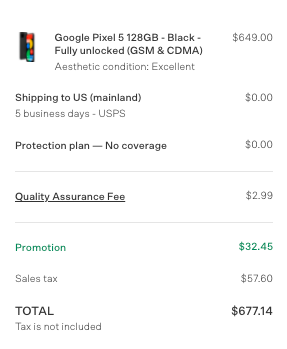The image depicts a screenshot of a shopping cart from an unidentified e-commerce site. The view shows items being purchased, likely on a digital device, although it is unclear whether it is a laptop, desktop, cell phone, or tablet. 

At the top left of the cart, there is an image of a phone, identified by its distinct black cover. The screen displays a design with a red area, a light blue or bluish-green patch, a yellow patch, a small red circle, and a small bluish-green circle, all identifying features of the Google Pixel interface.

The top of the text section indicates the item: "Google Pixel 5, 128GB, Black, Fully Unlocked GSM and CDMA." The phone's condition is described as "excellent." The price listed is $649. Shipping within the US mainland takes five business days via USPS and is free. No protection plan has been selected for the item.

Additional charges include a quality assurance fee of $2.99. A promotion discount of $32.45 has been applied. Sales tax amounts to $57.60, bringing the subtotal to $677.14, with tax included.